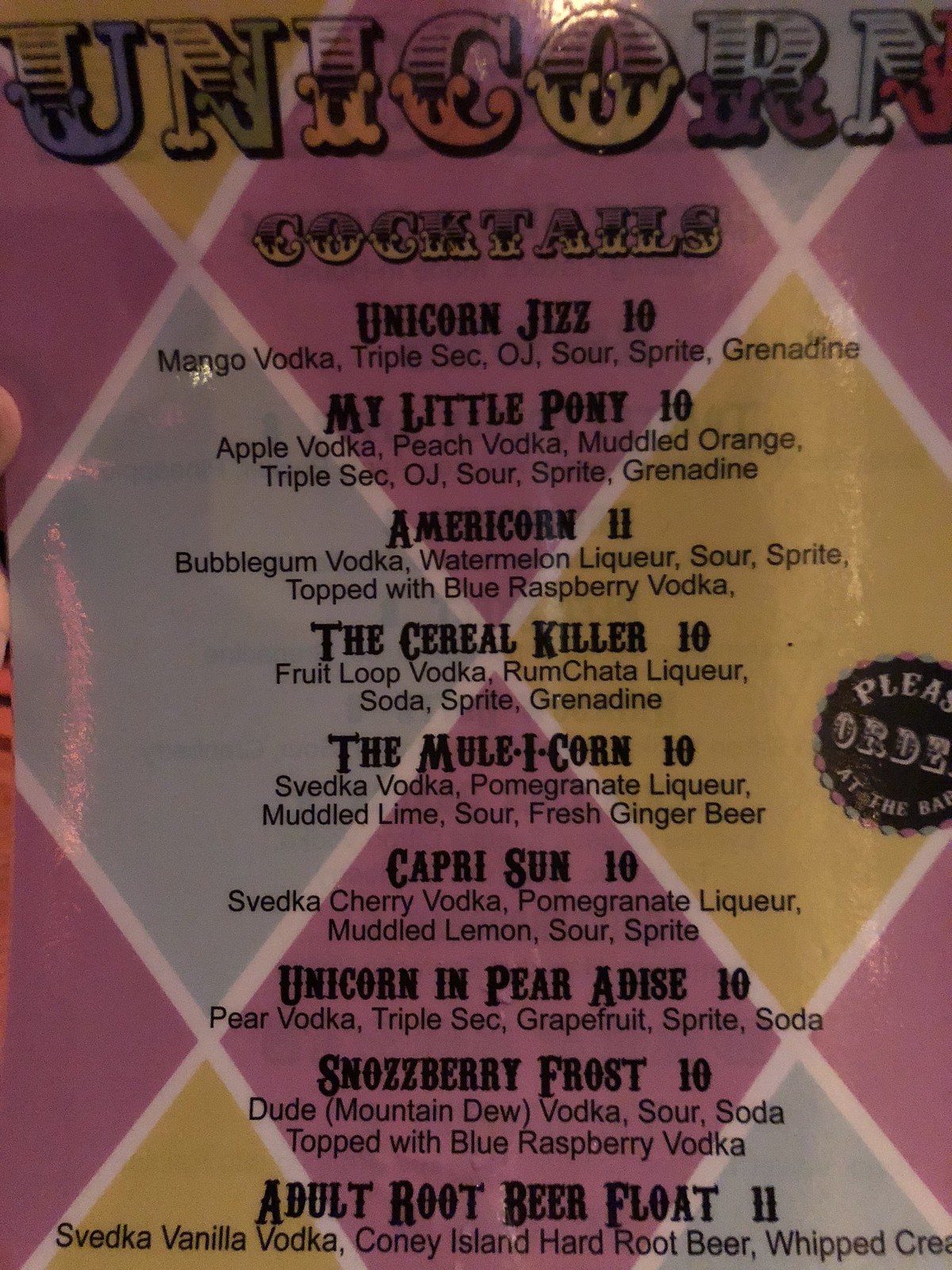This photograph showcases a vividly colorful and whimsically designed cocktail menu. The background is intricately patterned with diamonds of varying colors, primarily dark pink, interspersed with several light blue and yellow diamonds, all crisscrossed by white lines. 

At the top, the word "UNICORN" is emblazoned in ornate, multi-colored lettering. Directly below, in elegant yellow and black print, the menu declares "COCKTAILS." The first listed cocktail, titled "UNICORN JIZZ," is priced at 10 and described with its ingredients: MANGO VODKA, TRIPLE SEC, OJ, SOUR, SPRITE, and GRENADINE.

Following that, another drink called "MY LITTLE PONY," also priced at 10, is detailed with APPLE VODKA, PEACH VODKA, MUDDLED ORANGE, TRIPLE SEC, OJ, SOUR, SPRITE, and GRENADINE. 

Next on the list is the "AMERICORN," which costs 11 and includes BUBBLEGUM VODKA, WATERMELON LIQUEUR, SOUR, SPRITE, and is topped with BLUE RASPBERRY VODKA.

Lastly, "THE CEREAL KILLER," referred to playfully as "CEREAL WITH A C," is priced at 10 and features FRUIT LOOP VODKA, RUMCHATA LIQUEUR, SODA, SPRITE, and GRENADINE.

To the right middle of the menu, a round black medallion bordered in white prominently displays the message "PLEASE ORDER AT THE BAR" in clear white letters. The drink titles and components continue beyond the listed cocktails, offering a playful yet comprehensive array of colorful and creative options.